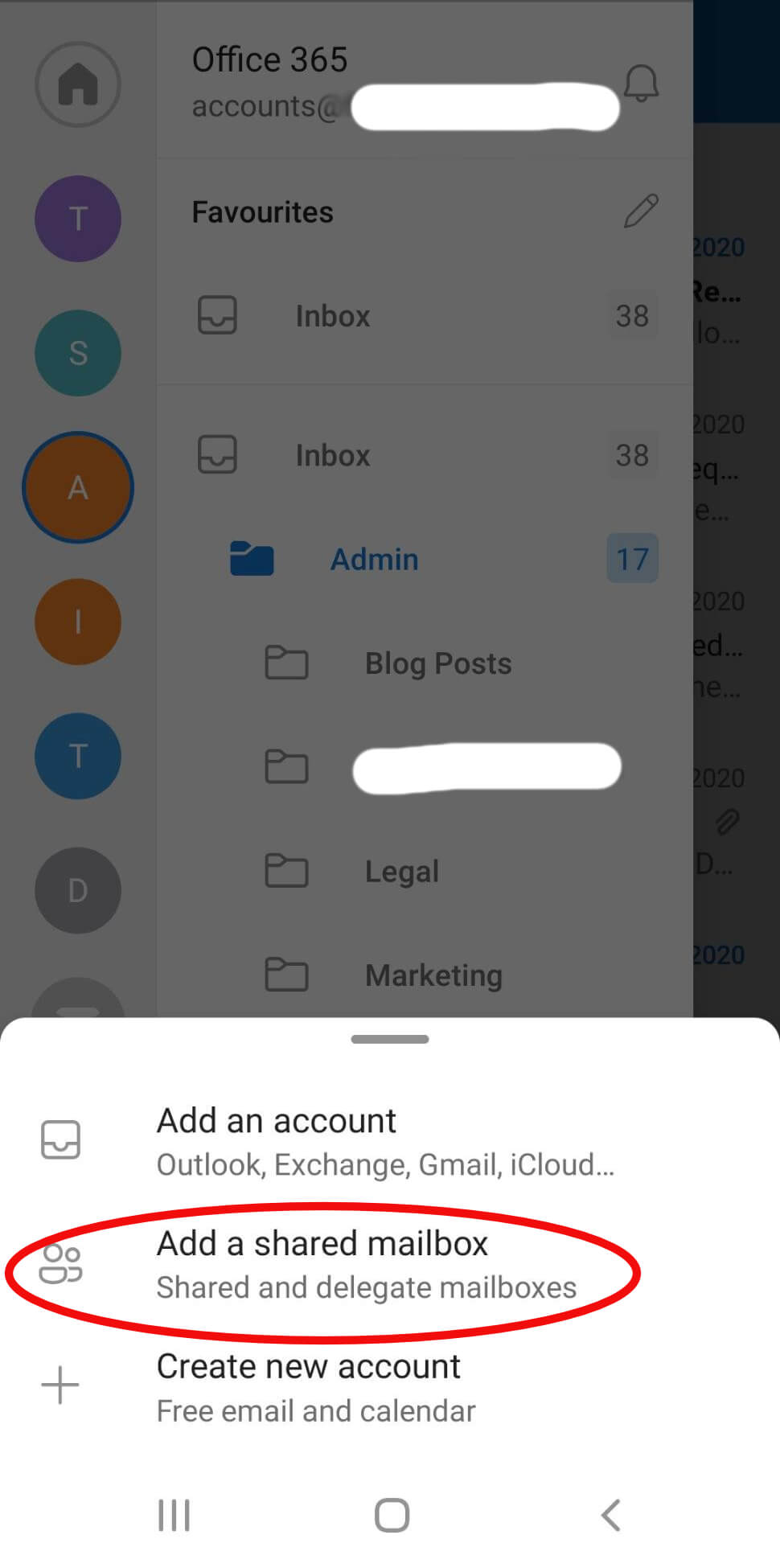The image is a detailed screenshot from a mobile email application, most likely Microsoft's Outlook. At the very top, it prominently displays the Office 365 logo alongside an email address, which has been partially blurred for privacy reasons. Following this, there is a section labeled "Favorites," which is indicated by an icon resembling a bar. Under this section, the "Inbox" is listed with a count of 38 unread emails.

Below the "Favorites" section, various folders are organized, including "Inbox" (38 unread emails), "Admin" (17 unread emails), "Blog Posts," "Legal," and "Marketing." On the right side of the screen, there are user avatars represented by initials—such as T, S, A, T, and D—likely corresponding to different individuals' names.

At the bottom of the screen, a navigation menu is visible, offering several options: "Add an account," "Add a shared mailbox," and "Create a new account." The "Add shared mailbox" option is circled in red, suggesting that the screenshot's purpose is to guide users on how to add a shared mailbox. This placement indicates that the screenshot is from the settings or account management section of the email app, neatly highlighting the option to add a shared mailbox for easy identification.